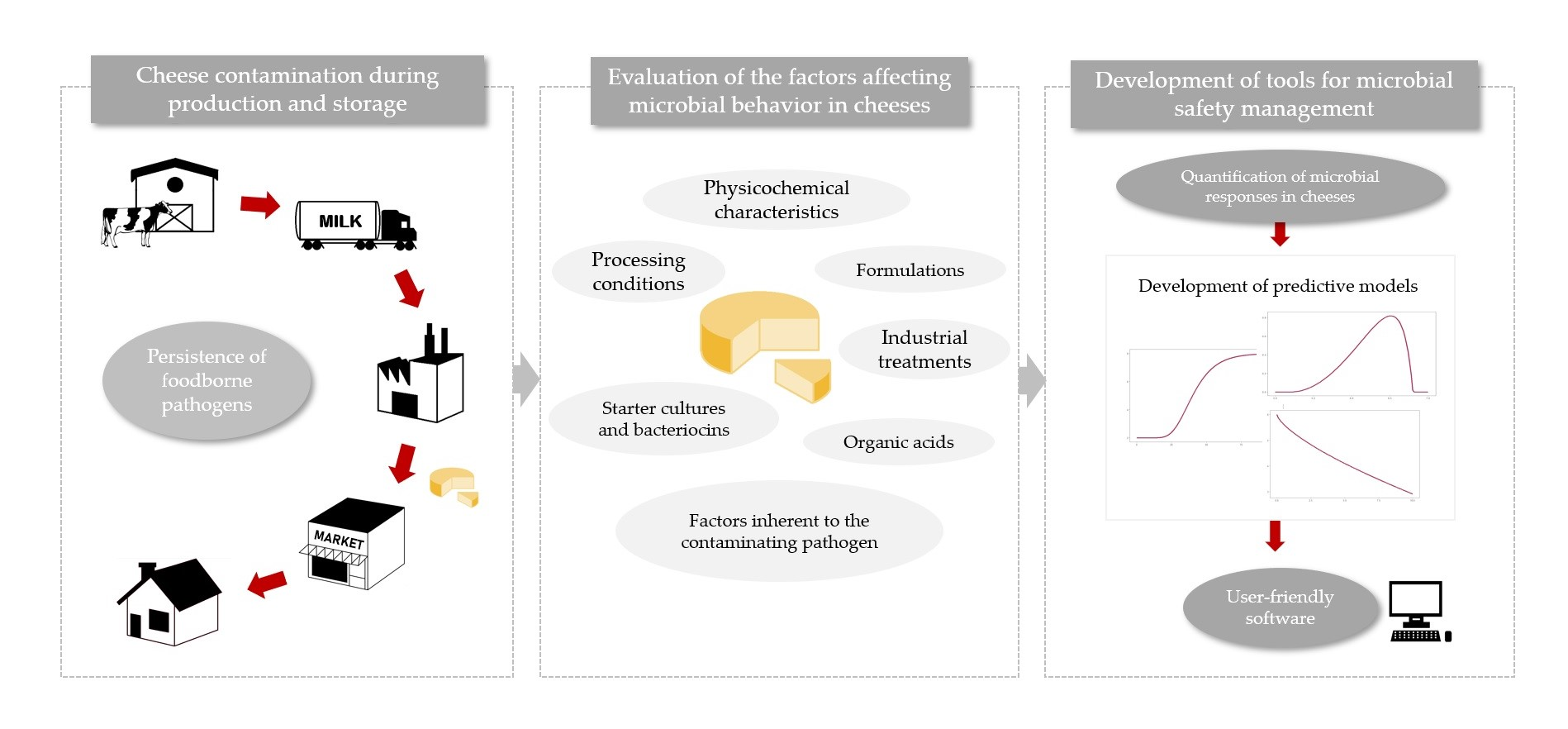The illustration is a scientific pictogram depicting the process of cheese contamination during production and storage. The image is divided into three vertical boxes, each containing detailed segments of the overall topic. 

The first box, titled "Cheese Contamination During Production and Storage," features images of a cow, a barn, trucks, a market, and a house, all interconnected with arrows to show the supply chain. It highlights the persistence of foodborne pathogens throughout this process with an emphasis on contamination points.

The second box, "Evaluation of the Factors Affecting Microbial Behavior in Cheese," is centered around a yellow cheese wheel with a wedge cut out. Surrounding the cheese are gray bubbles detailing various factors such as physiochemical characteristics, formulations, industrial treatments, organic acids, and contaminating pathogens that influence microbial behavior.

The third and final box, "Development of Tools for Microbial Safety Management," showcases a computer screen with graphs and a red curve above it. This section emphasizes the creation of tools for ensuring microbial safety in cheese, including user-friendly software for quantifying microbial responses.

Centrally placed gray ovals and arrows connect these boxes, illustrating the flow of information and processes between each stage in the cheese production and storage sequence.